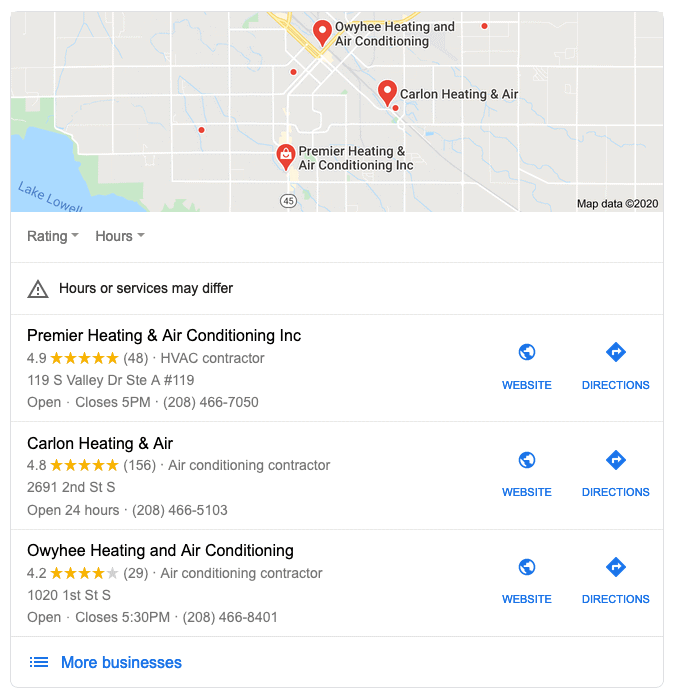The image presented is a Google Maps search result display for places related to Heating and Air Conditioning services. The overall background of the image is white, with a prominent rectangular box at the very top showcasing the key search information.

Underneath the rectangular box, the main visible area is the map highlighting three specific search results, with each location marked by distinct red pins. Below the map, detailed information about these locations is provided:

1. **Premier Heating and Air Conditioning Inc.**
   - **Rating:** 4.9 stars based on 48 ratings.
   - **Category:** HVAC Contractor.
   - **Status:** Currently open, closes at 5:00 PM.
   - **Contact Information:** Address provided with a phone number.
   - **Additional Options:** Icons for website access and directions are available.

2. **Garland Heating and Air**
   - **Rating:** 4.8 stars based on 156 reviews.
   - **Status:** Open 24 hours.
   - **Contact Information:** Address provided with a phone number.
   - **Additional Options:** Icons for website access and directions are available.

3. **Aohi Heating and Air Conditioning**
   - **Rating:** 4.2 stars based on 29 reviews.
   - **Status:** Currently open, closes at 5:30 PM.
   - **Contact Information:** Address provided with a phone number.
   - **Additional Options:** Icons for website access and directions are available.

Beneath the listing of these search results is a disclaimer stating that operating hours or services may differ, ensuring users are aware of potential variations.

At the very bottom, written in blue text, there is an option to see more businesses related to the search, offering users further exploration of additional service providers.